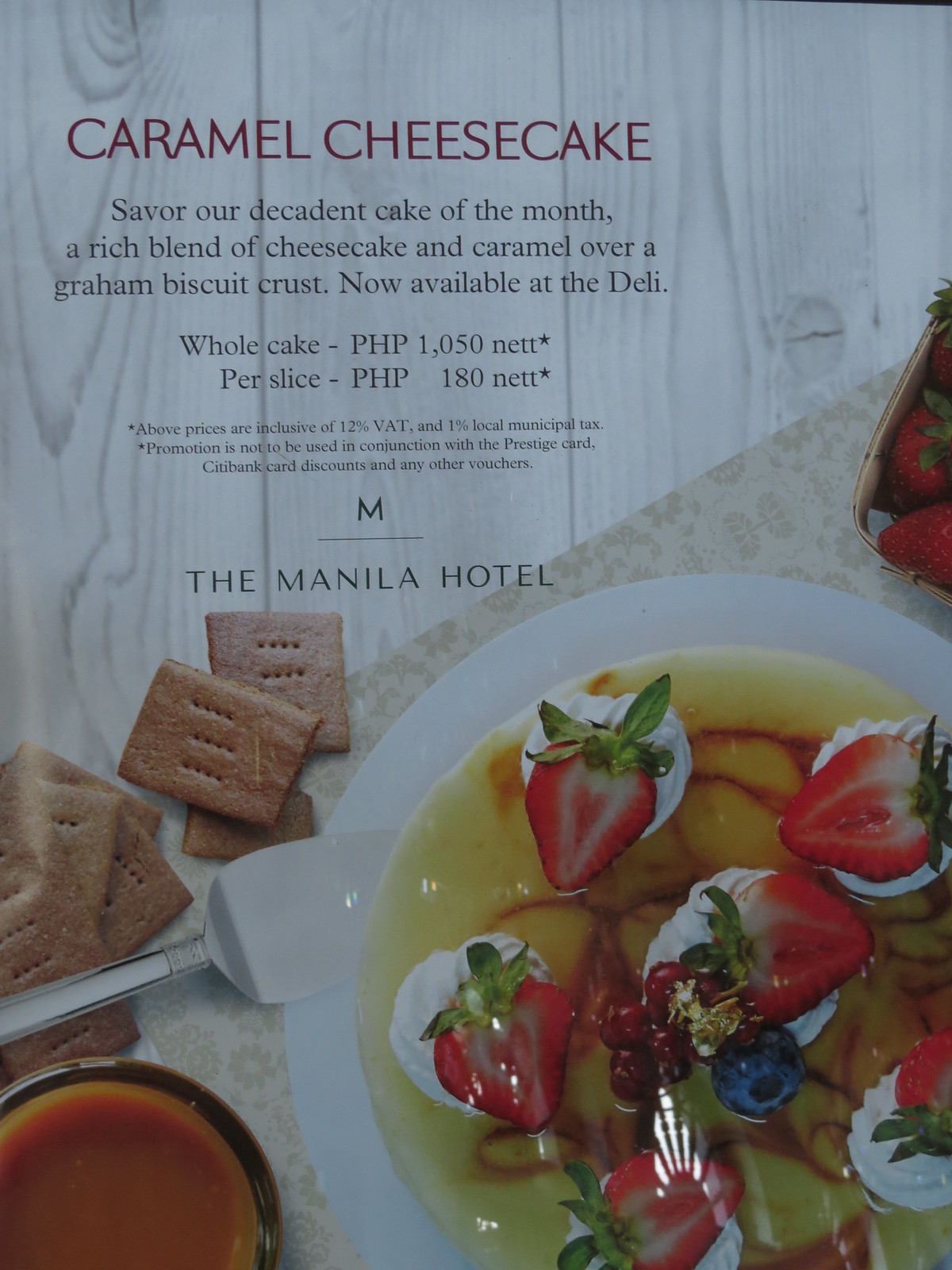The image is a magazine advertisement for the Manila Hotel, showcasing their Caramel Cheesecake as the "cake of the month." The cheesecake, presented on a white plate with a silver serving knife, is topped with a caramel glaze and adorned with dollops of whipped cream. Sliced strawberries with their leaves still attached, blueberries, and small red berries are artfully placed on top of the whipped cream. In the lower left corner, there's a small glass bowl filled with caramel sauce, and nearby, assorted cookies or biscuits are scattered. The plate rests on a textured fabric atop a white wooden table. On the right side, a wicker basket filled with strawberries is partially visible. The promotional text reads: "Caramel Cheesecake. Savor our decadent cake of the month, a rich blend of cheesecake and caramel over a graham biscuit crust, now available at the deli. Whole cake PHP 1050 net, per slice PHP 180 net. Prices are inclusive of 12% VAT and 1% local municipal tax. Promotion is not to be used in conjunction with the Prestige Card, Citibank card discounts, or any other vouchers." Completing the ad, the Manila Hotel logo, represented by an underlined 'M,' is prominently featured.